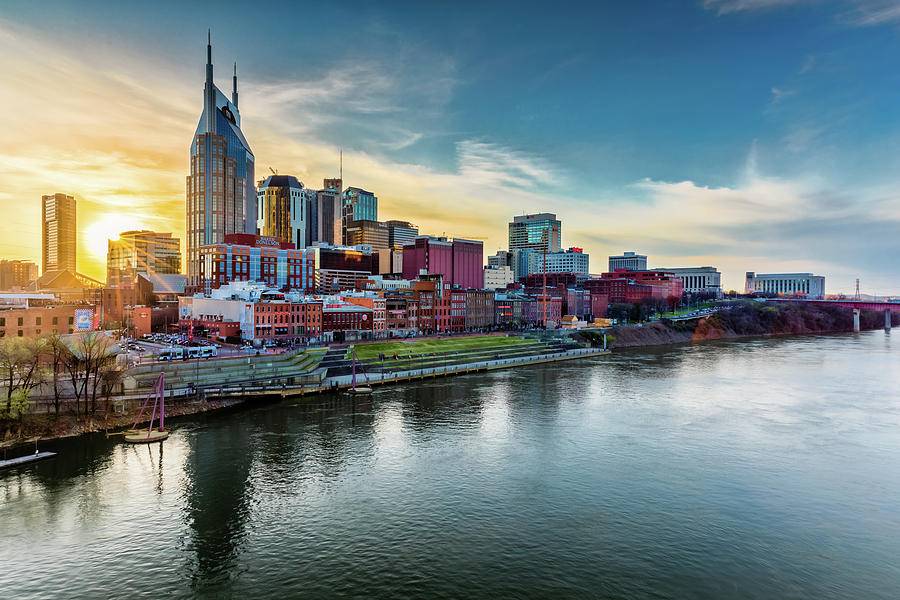The image depicts a city waterfront during either sunrise or sunset, with a vibrant and colorful skyline. Dominating the skyline is a prominent skyscraper on the left, distinguished by its rounded walls and two sharp spires reaching skyward. The sky transitions from a darker blue to a brilliantly lit yellow hue where it meets the bright orange sun near the horizon, casting a warm glow across the scene. Below, the calm waters of a large river reflect the city's palette, shifting from a dark blue to a light green near the shore. The waterfront boasts a series of stairs ascending from the river's edge, covered in patches of green grass, leading up to densely packed buildings of varying heights and vivid colors including oranges, pinks, blues, and purples, possibly accentuated by the sunlight. In the distance on the right, a bridge with a blue railing and a pink underside spans the river, adding to the picturesque quality of the cityscape. There are no visible people, giving a peaceful, almost surreal feel to the scene.